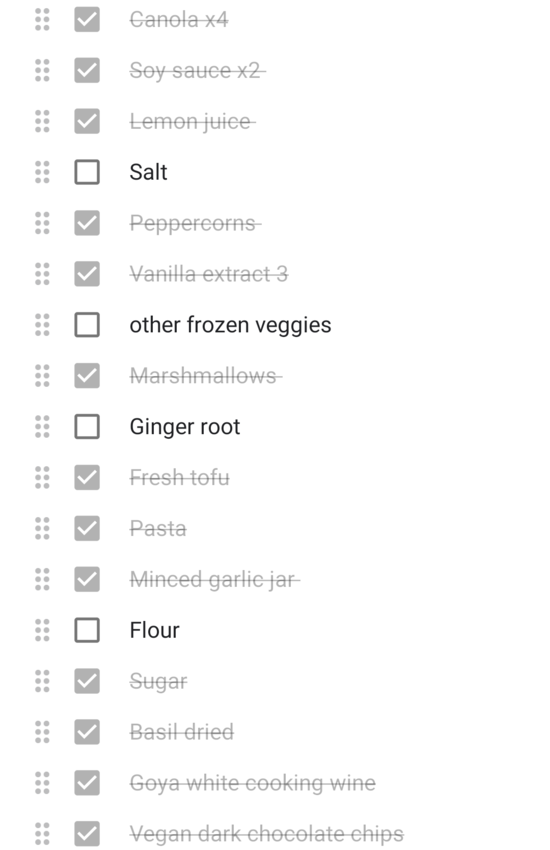This image is a detailed screenshot of a grocery list displayed on a cell phone with a white background. The list features items that have been segmented based on their purchase status. 

The items that have been purchased are rendered in light gray text with a line through them and a checkmark in front. These include:
- Canola (4 times)
- Soy Sauce (2 times)
- Lemon Juice
- Peppercorns
- Vanilla Extract (3 times)
- Marshmallows
- Fresh Tofu
- Pasta
- Minced Garlic Jar
- Sugar
- Dried Basil
- Goya White Cooking Wine
- Vegan Dark Chocolate Chips

Remaining items that have yet to be purchased are displayed in bold black text without a strikethrough or checkmark. These items include:
- Salt
- Other Frozen Veggies
- Ginger Root
- Flour

To the left of each grocery item, there is a set of six dots arranged in two vertical lines of three (similar to a drag handle), allowing users to click and drag items up or down to rearrange the list according to their preference.